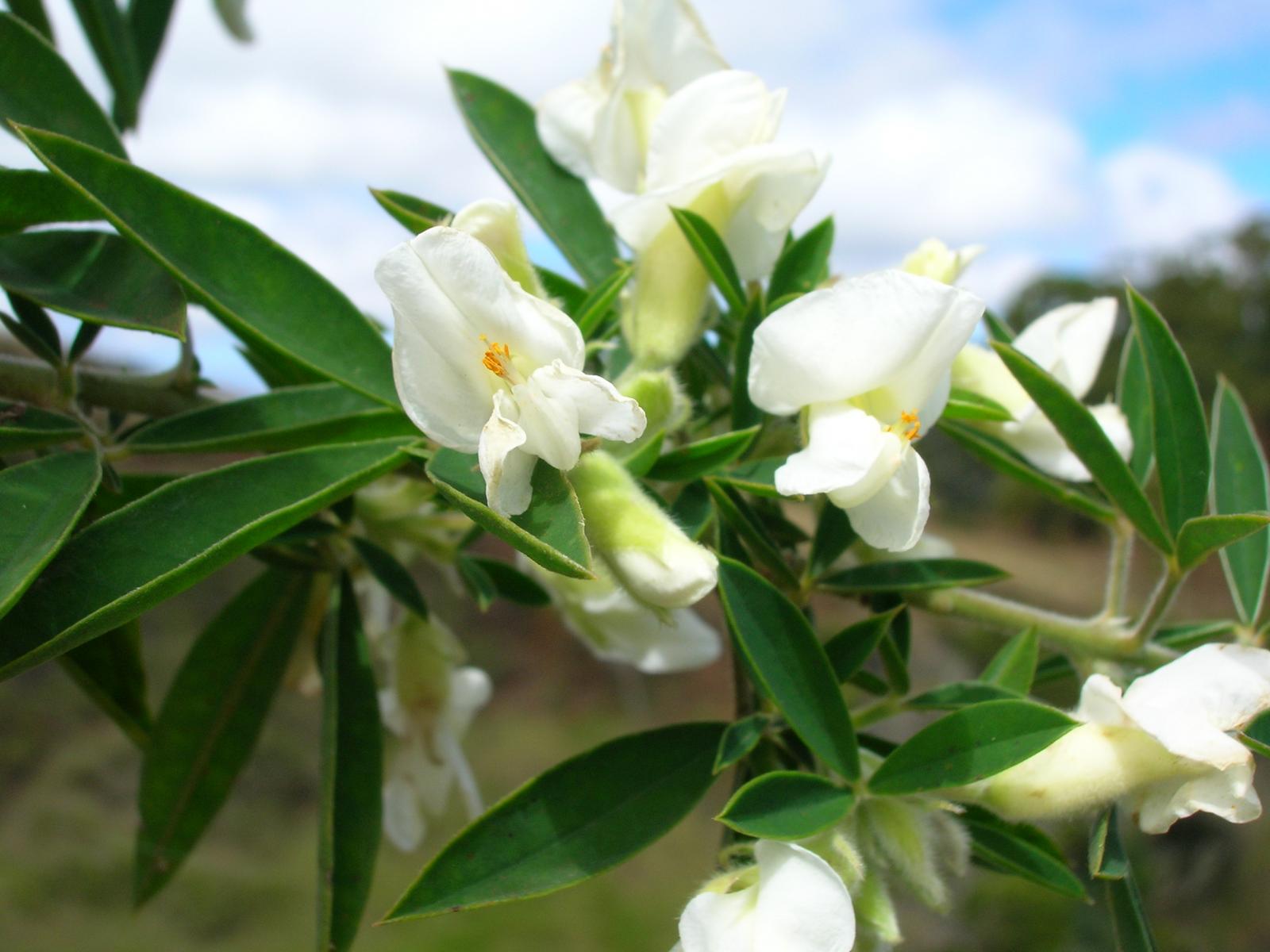In this outdoor landscape-oriented photograph, we observe a close-up of white flowers with light yellow accents, likely resembling orchids or irises. The primary focus reveals these intricate flowers, characterized by upright petals at the back and folded petals at the front, along with conspicuous stamens in the center. Surrounding the flowers are deep green, narrow, oblong leaves, seemingly longer than the flowers themselves.

The image also captures several flower buds, distributed across the scene, with some at the bottom and others to the left, waiting to bloom. The flowers and leaves are supported by light green stems. In the blurry background, grassy patches and dark green trees are faintly visible, framed against a sky that appears mostly cloudy with sparse glimpses of blue, indicating a bright daytime setting. The notable blur emphasizes the main flowers and leaves, enhancing their vivid details against a softly diffused backdrop.